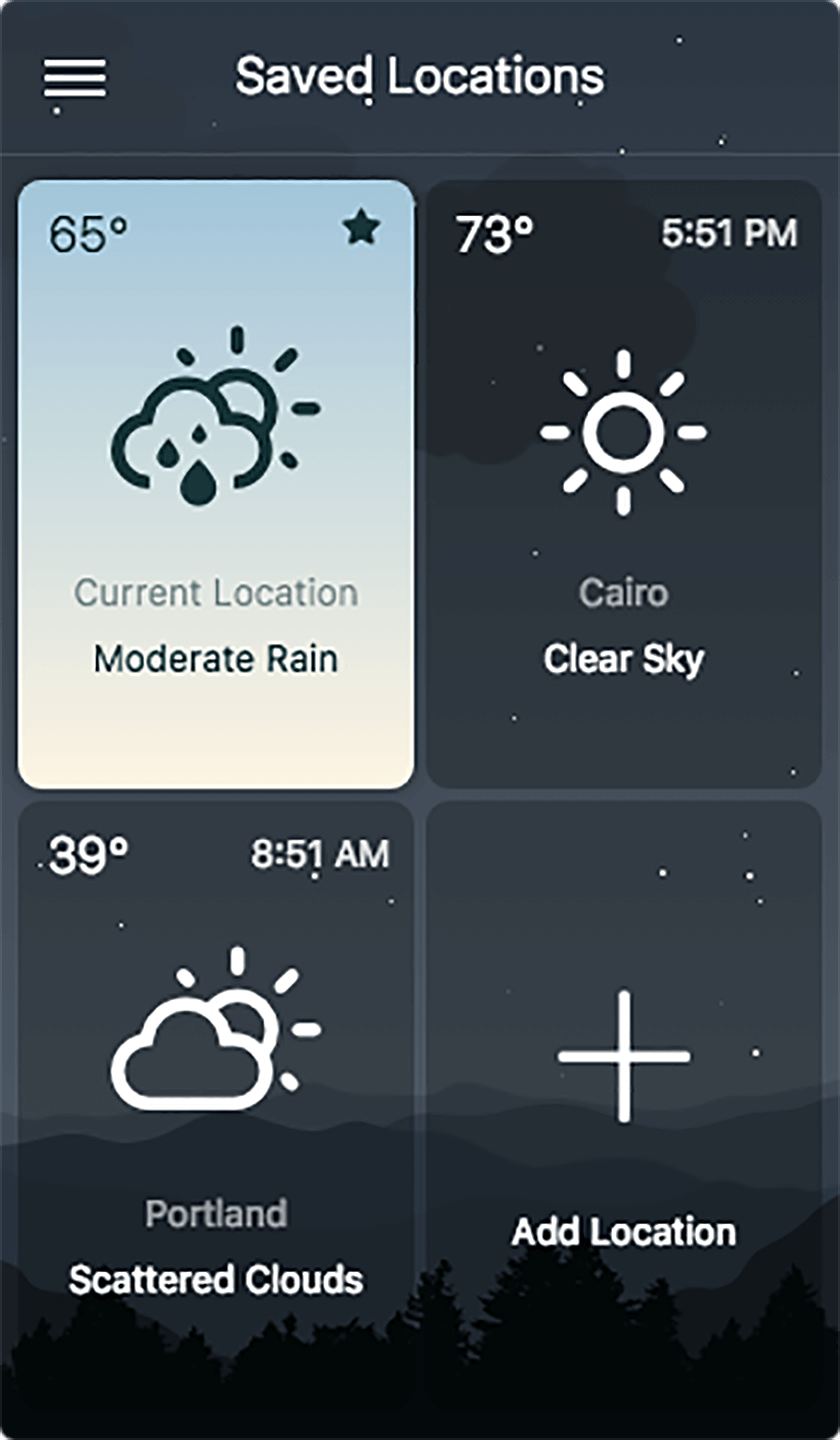Image Description:

The image portrays a multi-layered user interface set against a backdrop of a starry sky with a faintly visible mountainous region and trees at the bottom. The background is slightly transparent, displaying various overlays from an app.

In the upper left corner, there are three white lines indicating an expandable menu. Centered in bold white text is the label "Save to Locations". Below this are four rounded-rectangle sections each offering different information.

The top-left rectangle features a gradient background transitioning from light blue at the top to off-white at the bottom. At the upper left, the temperature reads "65 degrees" in rounded, black, sans-serif font. To the right, there's a filled black star icon. The central area of this section depicts an outline of a cloud with three raindrops of varying sizes, from largest to smallest: bottom, left, and behind. Additionally, there’s an outline of a sun with five rays. Below these icons, the text "Current Location" appears in light blue, and "Moderate Rain" is written in a darker color.

The top-right rectangle maintains a transparent background. Upper-left text reads "73 degrees" in white, while to the right, it states "5:51 PM" also in white. Below, a sun icon with several rays is displayed. The location "Cairo" is listed in light gray, with the weather condition "Clear Sky" beneath it in white.